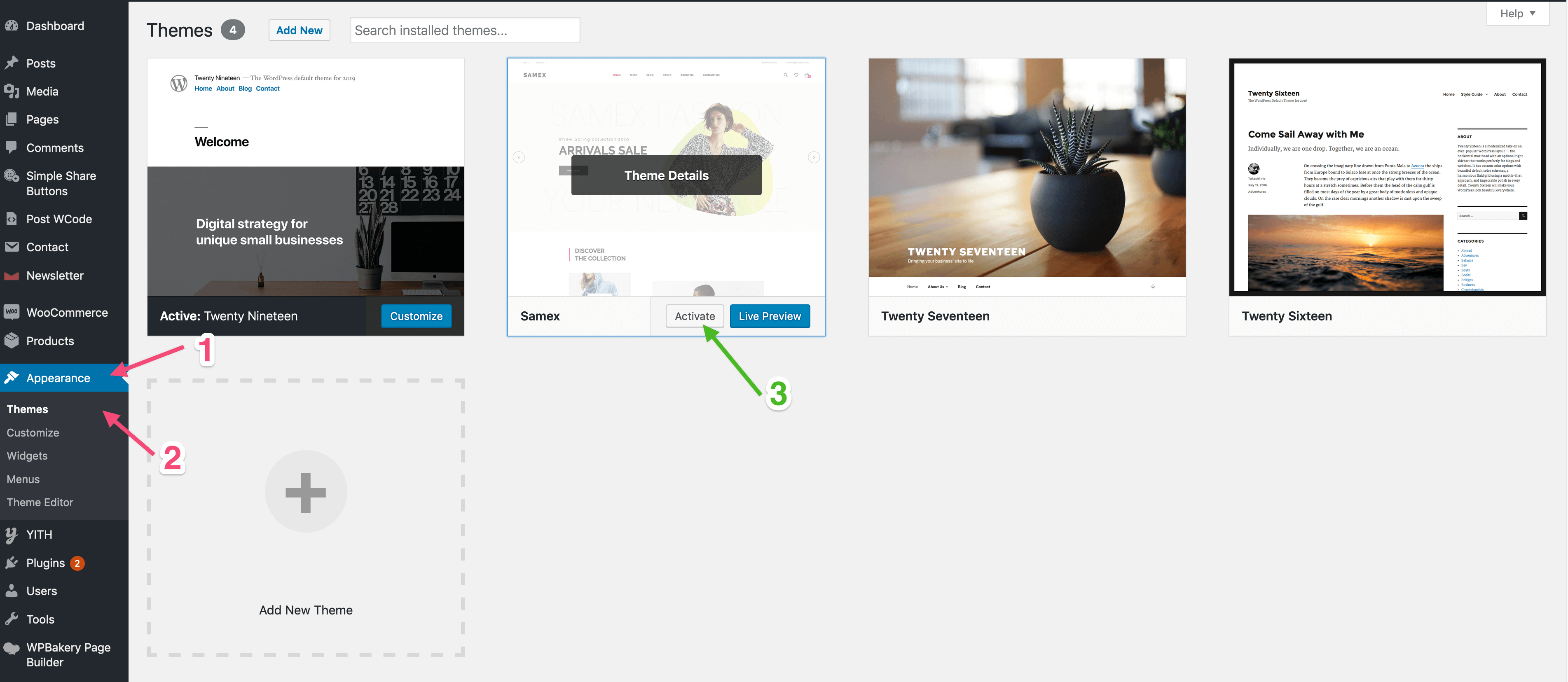The image showcases the WordPress website builder interface. On the left, a dark grey menu provides various options such as Dashboard, Posts, Media, Pages, Comments, Simple Shape Button, Post, WCode, Contact, Newsletter, WooCommerce, Products, Appearance, Plugins, Users, Tools, and WPBakery Page Builder. The 'Appearance' section is currently expanded, revealing sub-options including Themes, Customize, Widgets, Menus, and Theme Editor.

Annotations guide the viewer through a step-by-step process for changing the website theme. A pink "1" annotation points to 'Appearance,' indicating the first step. A pink "2" arrow directs to 'Themes,' showing the next step. A green "3" arrow points to the 'Activate' button on the second theme, which is the final step in the process.

On the right side of the image, under the 'Themes' section, there are four theme options displayed. The current active theme is titled "Welcome Digital Strategy for Unique Small Business" (Active 2019). Below it is the theme meant to be selected next, which corresponds to the green "3" annotation. The other themes are "2017," "Come Sail Away with Me," and one unnamed theme. A partition labeled "8 new" is also visible, along with a search bar that says "Search Installed Theme."